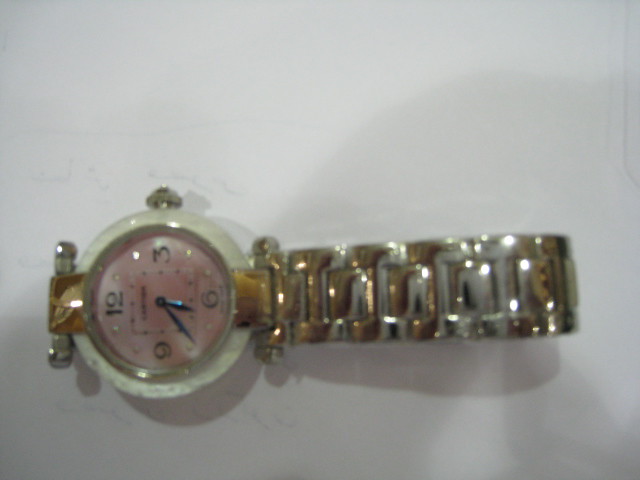This image depicts a slightly blurry photograph of a wristwatch displayed on a white background, giving the impression it is floating. The watch is oriented horizontally, with its top facing left and the band extending to the right. The band is a thin mix of gold and silver, resembling an elastic band, and leads to an oval watch face. The outer rim of the watch face has a white, slightly pearly tone, while the inner face exhibits an opaque pink color. Sparkly details suggest the presence of small diamonds. The watch features black hands indicating a time of 6:40. It includes numerical markers at 12, 3, 6, and 9, with dots marking the other hours. A silver dial is visible on the right side of the watch face, and the watch appears to be an analog, wind-up mechanism.